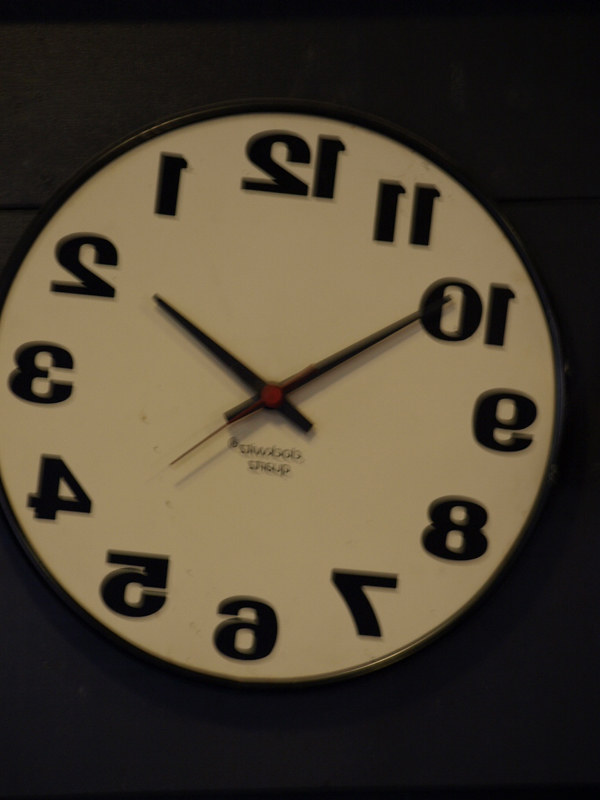This photograph features a slightly blurry image of a black-framed clock set against a dark gray background. The clock's white face showcases thick-font numbers that are reversed, adding an intriguing visual twist. It has two black hands for the hour and minute, and a contrasting red hand for the seconds. Black text, in a lighter shade, is subtly printed beneath the clock hands. Shadows from the clock and its hands are visible on the white face, enhancing the depth of the image. The background remains unobtrusive, allowing the clock to be the focal point, with no other objects in the frame.